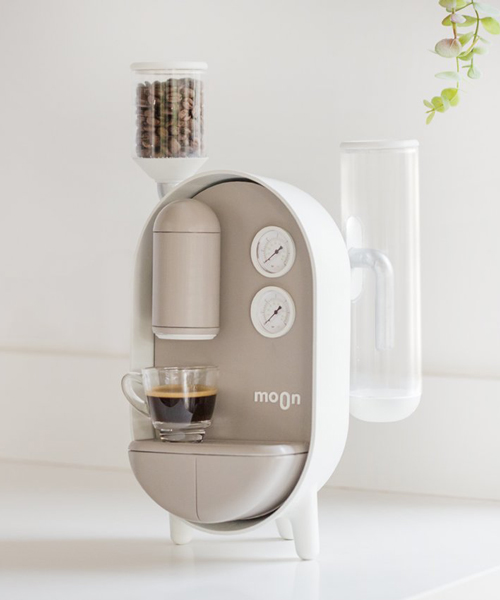The image showcases a sleek and futuristic white coffee machine positioned on a white countertop against a white background. The machine features an oval design with three small legs, giving it a modern and stylish appearance. To the right side of the coffee maker is a transparent water tank, while on the upper left side, there is a container designated for whole coffee beans, indicating the machine's built-in grinder capability. The front of the machine displays two round dials resembling clock faces and the brand name "Moon" beneath them within a brown section. This section also incorporates a shelf for placing a glass coffee cup, which is filled with a dark brown liquid topped with foam. The overall design includes curved elements and an intuitive layout, marking it as an innovative and advanced coffee-making appliance.